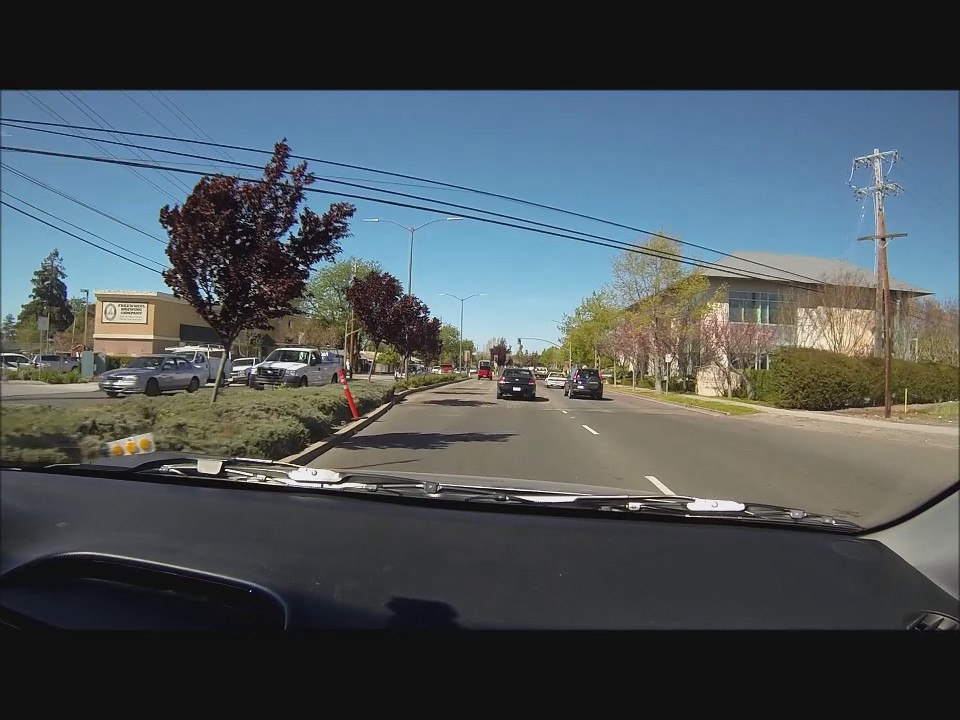This image captures a daytime scene in a town from the vantage point of a passenger in a car, looking out through the windshield. The dashboard of the car is black, contrasting with silver trim, suggesting it belongs to a silver car. At the bottom of the windshield, windshield wipers are visible. The clear, bright blue sky hints at a sunny afternoon, with no clouds in sight. 

Ahead stretches a light gray, four-lane divided roadway with white traffic lines, accommodating several other vehicles. On either side of the roadway, vibrant green bushes and reddish-leaved trees with skinny brown trunks line the street. To the left, there's a distant tan, square-shaped building, likely a business, though the sign is unreadable. On the right, a large tan building with several windows and a flat, trapezoidal-roof shingled in light gray stands prominently. Also visible are several tall, double-sided streetlights placed at intervals along the street. Black power lines crisscross the sky, adding to the urban landscape.